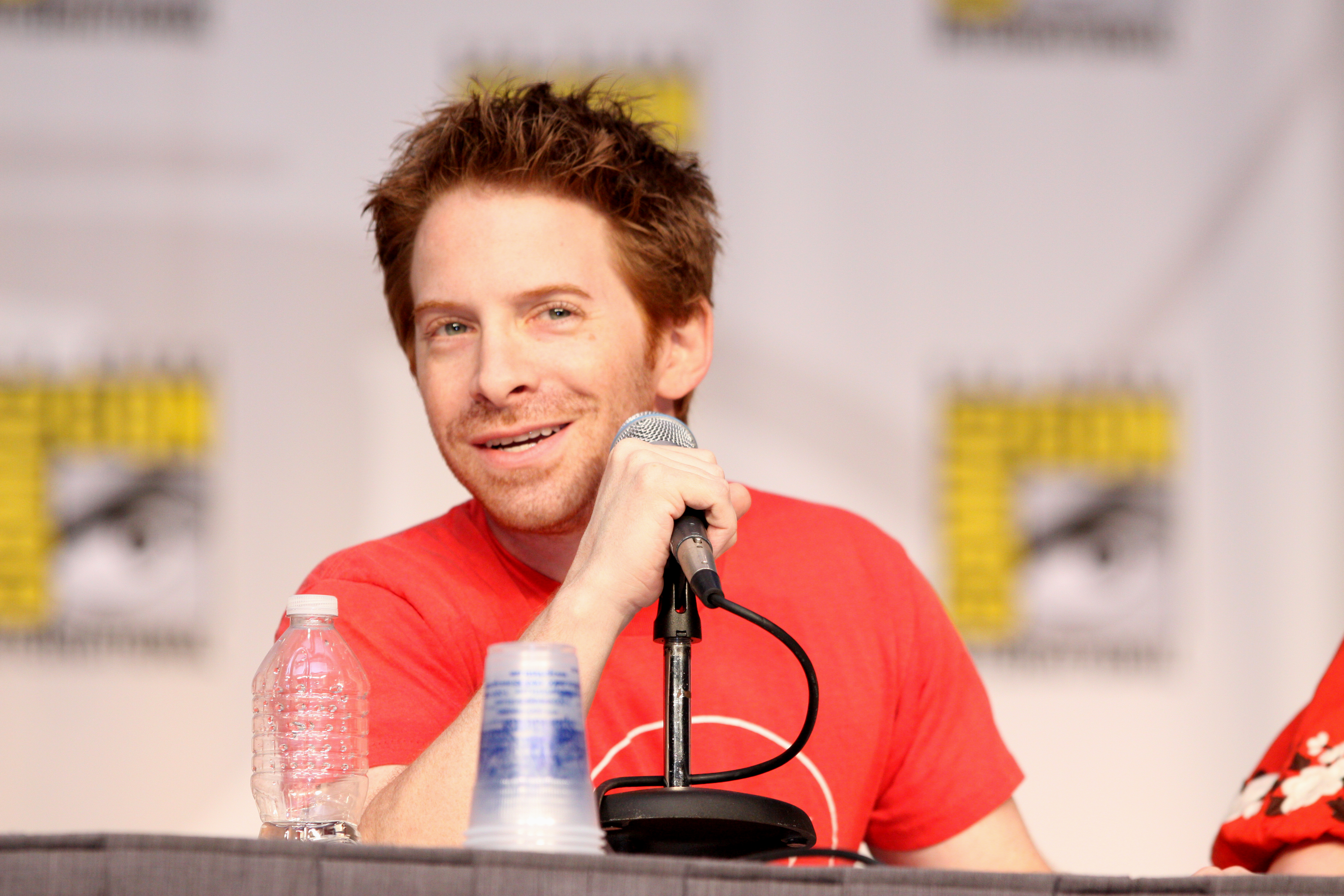In this color photograph, actor Seth Green is seated at a table adorned with a gray curtain tablecloth in the foreground. A clear, half-full plastic water bottle with a white cap sits on the table, accompanied by an upside-down stack of white plastic cups. In front of Seth is a silver microphone stand holding a microphone with a black base, from which a black wire extends below the table. Seth, sporting spiky reddish hair and a light stubble, is dressed in a short-sleeved red graphic t-shirt featuring a white circular line design. He smiles subtly while looking towards the top right corner of the photograph. The backdrop includes a discernible white wall covered with the Comic-Con logo, adding context to the scene. A hint of another person's red sleeve, decorated with white flowers and black leaves, peeks out on his right side.